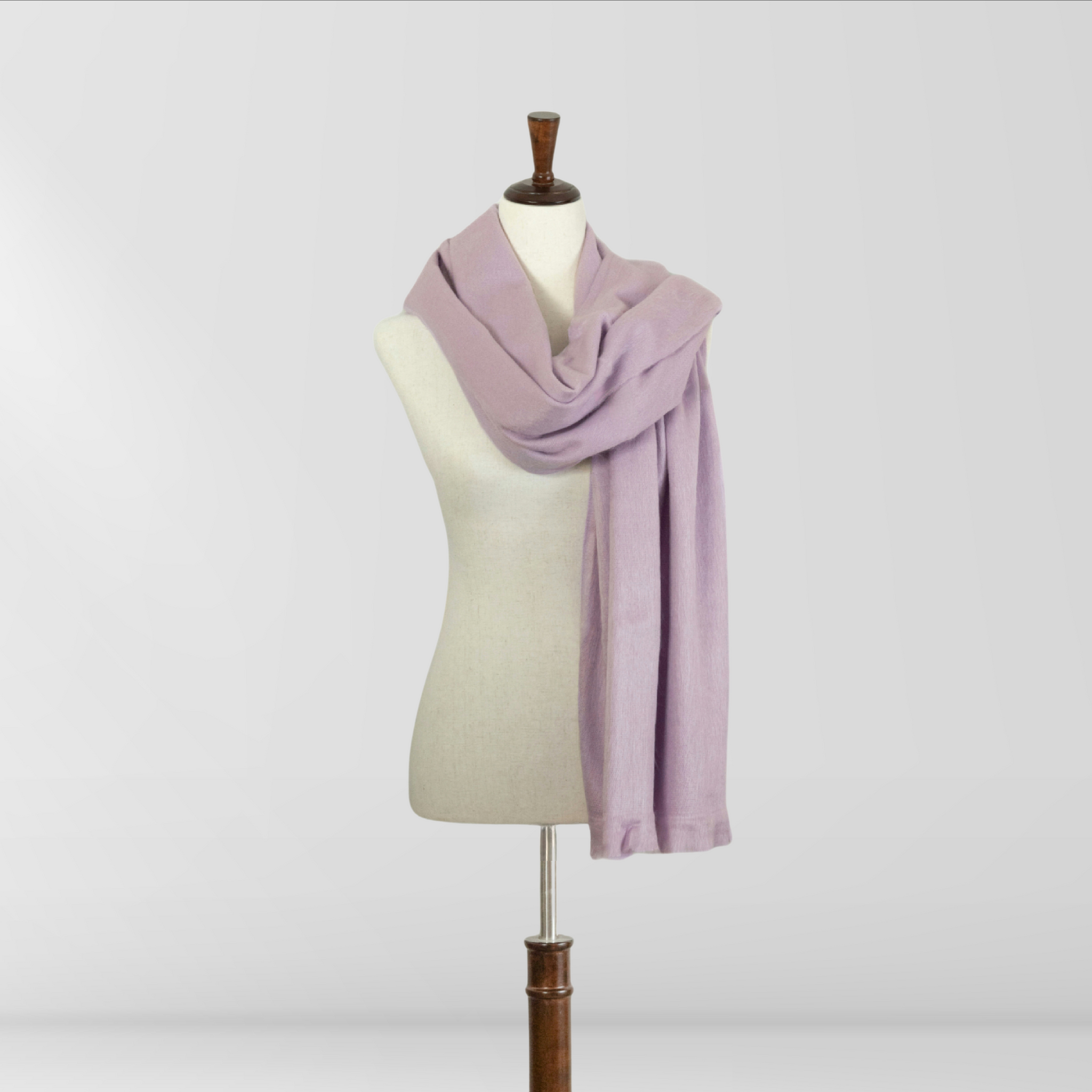This image features an off-white, headless, and armless dressmaker's dress form, designed to simulate a woman's torso. The dress form is elegantly mounted on an oak base, supported by a silver metal rod that extends through the torso and is capped with an oak knob at the neck. Complementing the minimalist aesthetic, a light pinkish-lavender or peachy-moth-colored scarf, likely made of soft flannel, is loosely draped around the neck. The scarf gracefully cascades down the right side of the form, while the rest of it wraps around and extends down the back, partially out of view. The background is stark white, enhancing the modern, sophisticated feel of the image. This dress form, with its finely curved torso, is clearly intended for fashion showcasing.